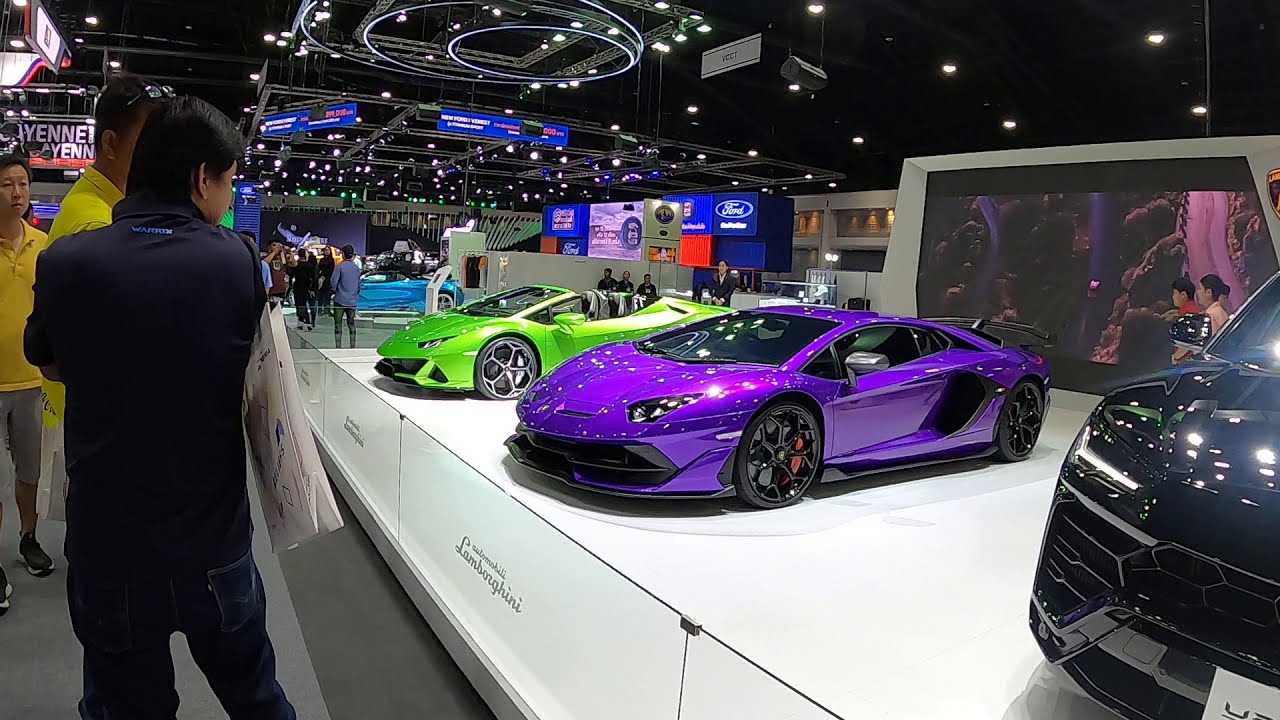This brightly lit and colorful indoor photograph captures a bustling car show. The image, horizontally rectangular without a border, prominently features about two and a quarter high-end sports cars on a white stage. In the foreground, a sleek purple Lamborghini and a vibrant green convertible Lamborghini are showcased, with the partial view of a black SUV on the side. Three men, two in yellow shirts and one in a dark blue shirt with blue jeans, are closely inspecting the cars, while others meander in the background. Overhead lights accentuate the reflective sheen of the vehicles' paint jobs. Visible logos, including Ford and others less discernible like Yemen, adorn the backdrop. The scene is filled with an array of fancy lighting and busy movement as attendees explore the array of displayed cars.